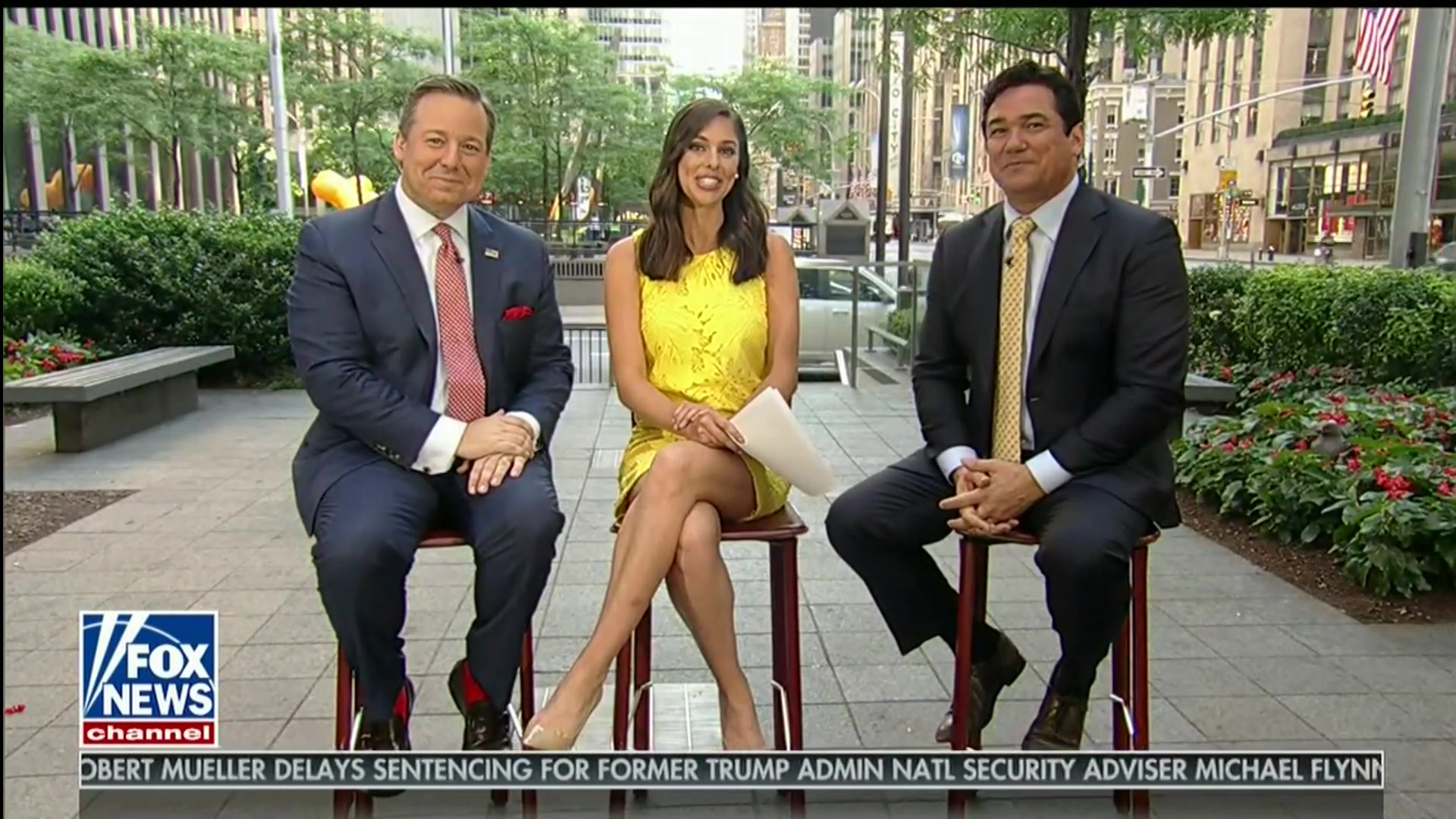The image is a screen grab of a Fox News program displayed on a TV, with a partially transparent banner at the bottom. The banner in white text reads, "Robert Mueller delays sentencing for former Trump administration National Security Advisor Michael Flynn." On the top left of this banner, a logo contains a blue square with a white border that reads, “Fox News” in white text with a blue border, and below that, in a red rectangle, “Channel” in white text. 

In the foreground, three news anchors are sitting on tall bar stools, facing the camera. The setting appears to be outside, featuring concrete square flooring. Behind the anchors are the bases of tall buildings, possibly skyscrapers, an array of trees, and an American flag hanging from a building in the upper right-hand corner.

On the left is an older white man in his 40s or 50s with slicked-back graying hair, dressed in a blue suit with a white shirt and a red tie. In the center sits a woman with shoulder-length brown hair, wearing a knee-length yellow dress and sitting with her legs crossed. To her right is another man, described as an older man possibly of Asian descent, in a black suit with a white shirt and a yellow tie.